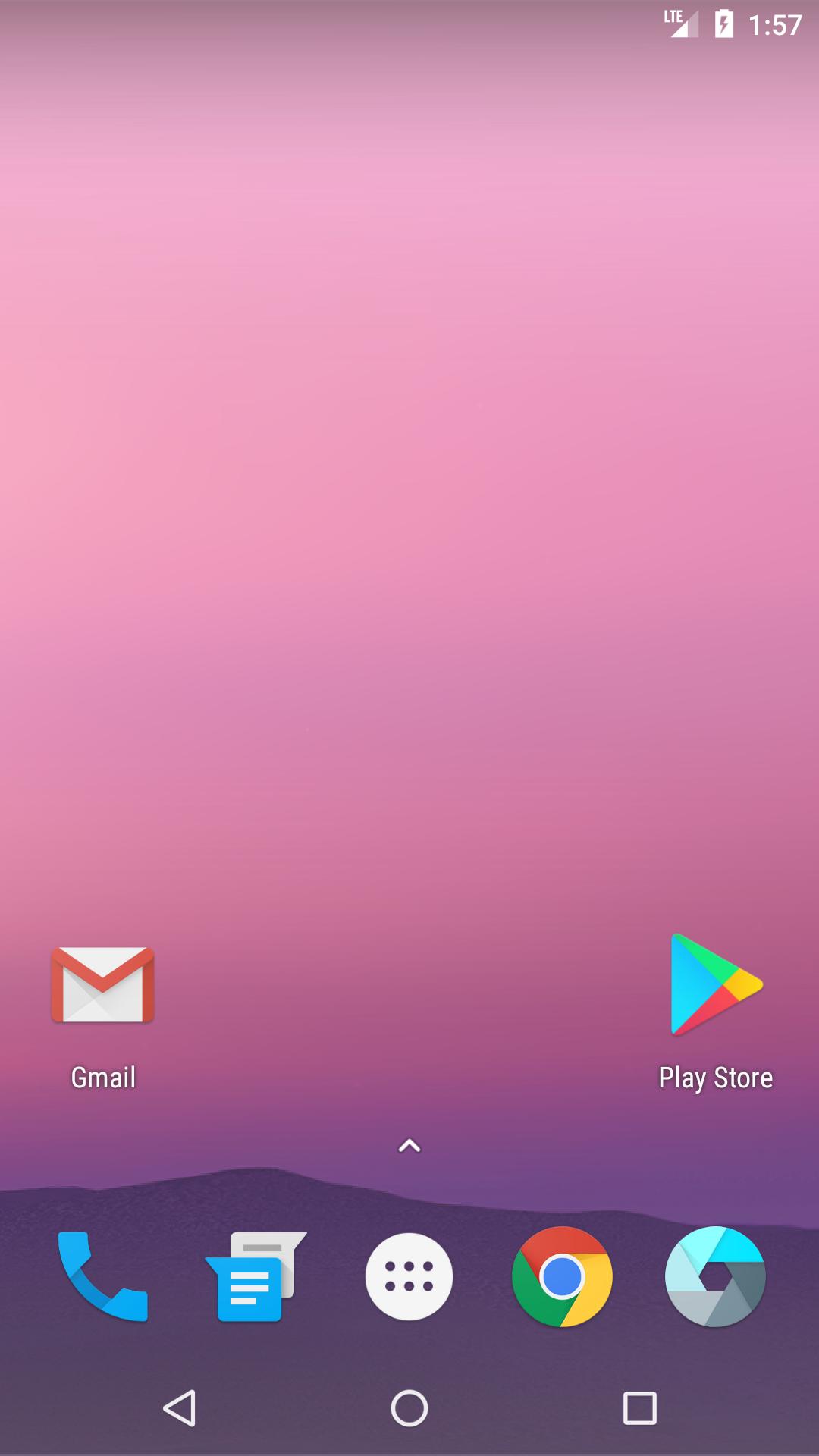This image depicts a smartphone home screen with a solid pink background, creating a minimalistic and somewhat surreal visual effect. The time displayed on the screen is 1:57, and the battery icon indicates a full charge. Prominently featured apps on the home screen include Gmail, Play Store, and Chrome, suggesting that this is an Android device. Despite the overall simplicity, a darker, abstract representation of a mountain range can be seen at the bottom of the background, adding a subtle contrast and a hint of depth to the otherwise stark layout. Overall, the image is unembellished and utilitarian, highlighting everyday digital tools against a uniquely colored backdrop.